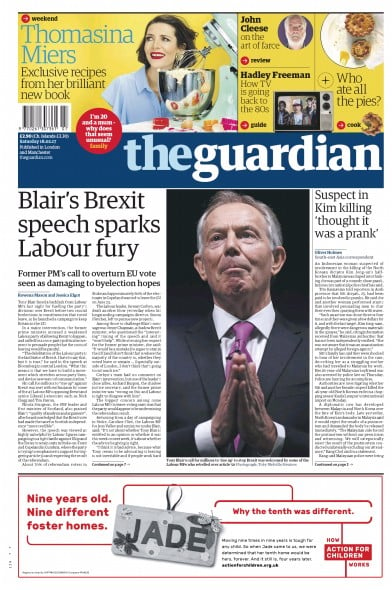This is an image of The Guardian's cover. At the top of the cover, there are two gold circles. The first circle contains an image of a brunette woman with striking red lipstick, dressed in a blue shirt, posing with a vintage light blue stand mixer that gives a 1950s vibe. There is some food visible near the mixer. Text in a mixture of blue and black reads, "Thomasina Meyer's exclusive recipes from her brilliant new book."

Below this circle, there is a white and black barcode, accompanied by some white text. Next to this barcode, there is a red circle with white text inside. Below these elements are a series of small images and blurbs. The first blurb, in black text, features "John Cleese on the art of farce" alongside a picture of John Cleese.

Next, there is an image of a plate with a baked good and a larger pie, accompanied by the text, "Who ate all the pies?" Following this, another blurb reads, "Hadley Freeman: How TV is going back to the 80s," alongside a gray old-school television displaying an image that looks like a scene from "Stranger Things."

Further down, a blue box contains the title "The Guardian." The prominent headline in the box is "Blair's Brexit speech sparks Labour fury," with the subheading, "Former PM's call to overturn EU vote seen as damaging to by-election hopes." An image of a politician with gray hair, wearing a white shirt, purple tie, and a navy coat, accompanies the article.

Another headline reads, "Suspect in Kim Killing thought it was a prank," followed by article text. At the bottom of the cover, there is an advertisement with a white background and red text that states, "Nine years old, nine different foster homes," followed by an image of a tag necklace labeled "Jade." The text below reads, "This is why the 10th was different," followed by a paragraph detailing how Action for Children made a difference.